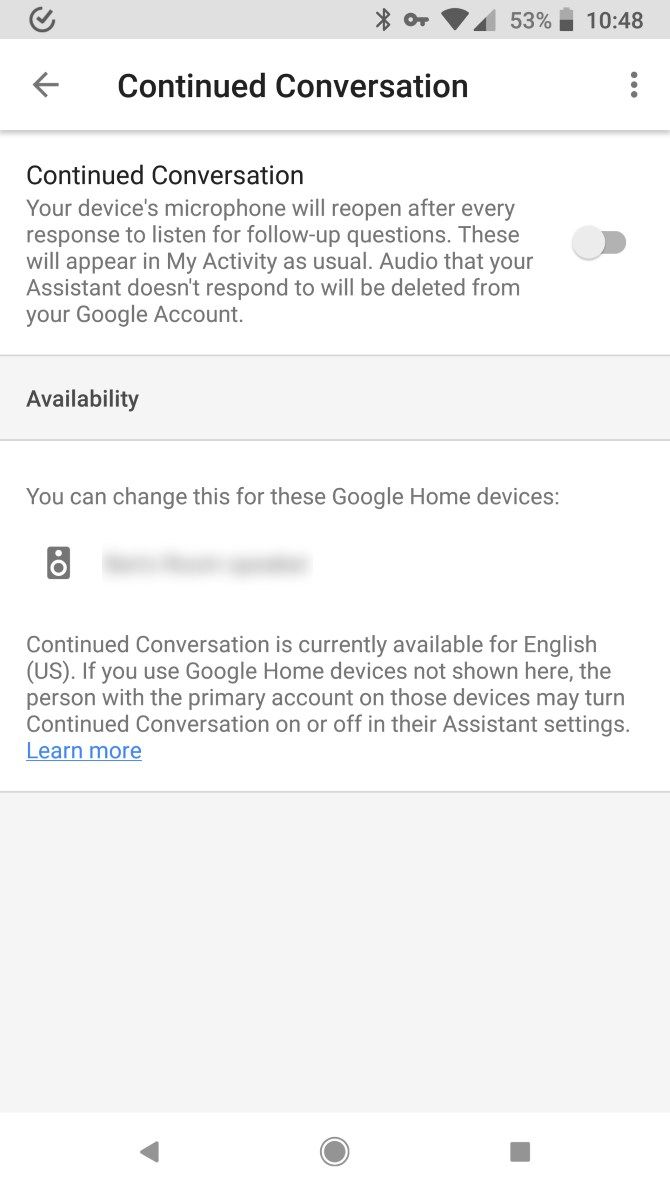The image displays a smartphone interface featuring several characteristic icons at the top, including the battery status and the time. Additionally, a prominent checkmark is visible in the top-left corner of the screen. Below these, bold black text reads "Continued Conversation," accompanied by a leftward-pointing arrow.

Further down, another "Continued Conversation" heading is followed by a detailed paragraph explaining that the device's microphone will reopen after each response to listen for follow-up questions, with this activity appearing in "My Activity" as usual. The paragraph also notes that any audio not responded to by the Google Assistant will be deleted from the user's Google account.

Adjacent to this paragraph is a grayed-out button, indicating it is currently inactive. Below this section, there is a heading labeled "Availability," which mentions altering settings for specific Google Home devices. Although one device is listed, its details are blurred, rendering them unreadable. To the left of this listing is a gray icon resembling a ring.

The text further clarifies that "continued conversation" is available exclusively in English (U.S.). It provides additional information on managing these settings, noting that the primary account holder on other Google Home devices may toggle this feature on or off in their Assistant settings.

Lastly, the screen features a "learn more" link, highlighted in blue, followed by an empty gray space, and concludes with three standard navigation icons at the bottom of the smartphone interface.